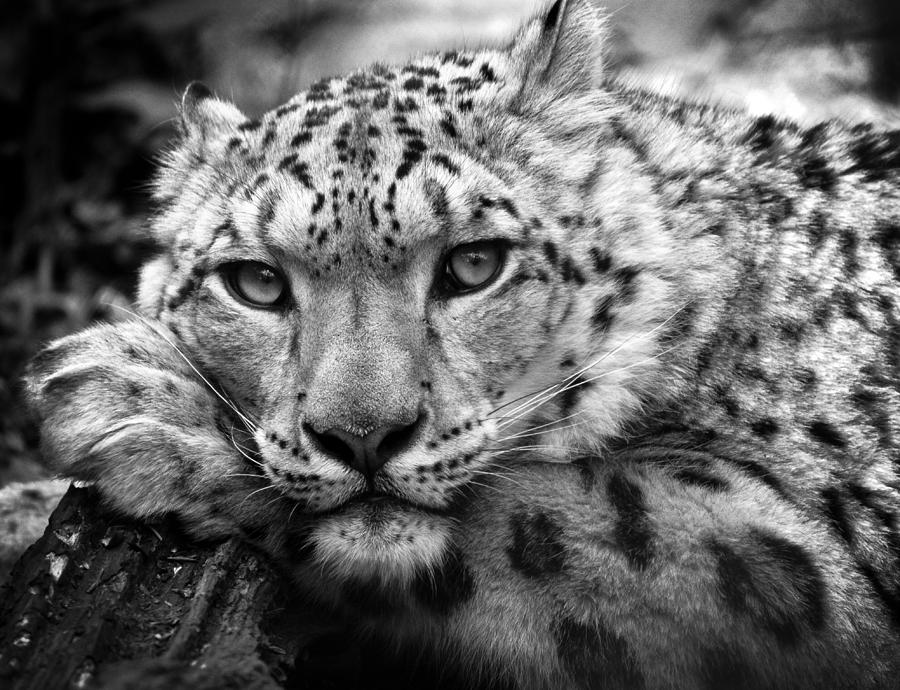This is a black and white close-up photograph of a leopard, capturing its head, upper back, shoulder, and one paw. The leopard, with its beautiful and captivating face, is reclining and has positioned its head on its left paw, which rests on what appears to be a fallen log or piece of rotten wood. The photograph showcases the leopard's striking spots, which vary in size and pattern across its forehead, forearms, and furry shoulders. Its ears are in different positions: the right ear is perked up while the left ear rests downward. The leopard's thin white whiskers emanate from black-dotted areas around its wide nose, and its shiny, expressive eyes seem to stare knowingly into the camera, giving an impression of a perfectly timed pose. The background is blurred with unidentifiable details, likely consisting of plants, emphasizing the leopard as the stunning focal point of this expertly captured image.